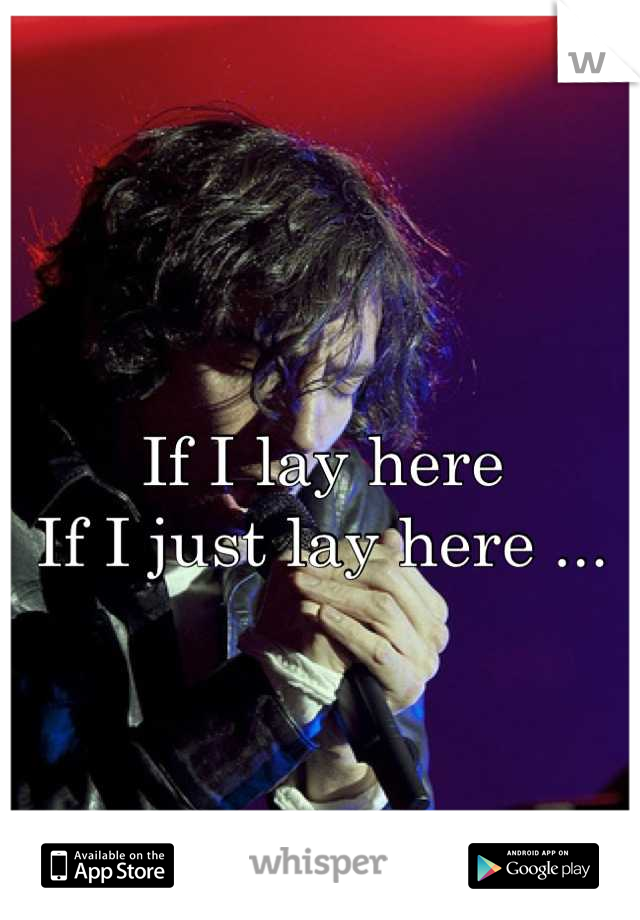The poster depicts a younger man with slightly unkempt hair huddled in his layered jacket, hands clasped. The background transitions from a deep brick red near his head to a purple-blue gradient. Prominently displayed in white uppercase and lowercase letters are lyrics: "If I lay here, if I just lay here..." This line is from a song by Snow Patrol. At the top of the poster is a large "W", and at the bottom, the word "Whisper" is shown along with mentions of the App Store and Google Play Store, indicating that it may be an advertisement for the Whisper app. The overall sense of the image and its text suggests a melancholic, reflective mood akin to the song's theme.